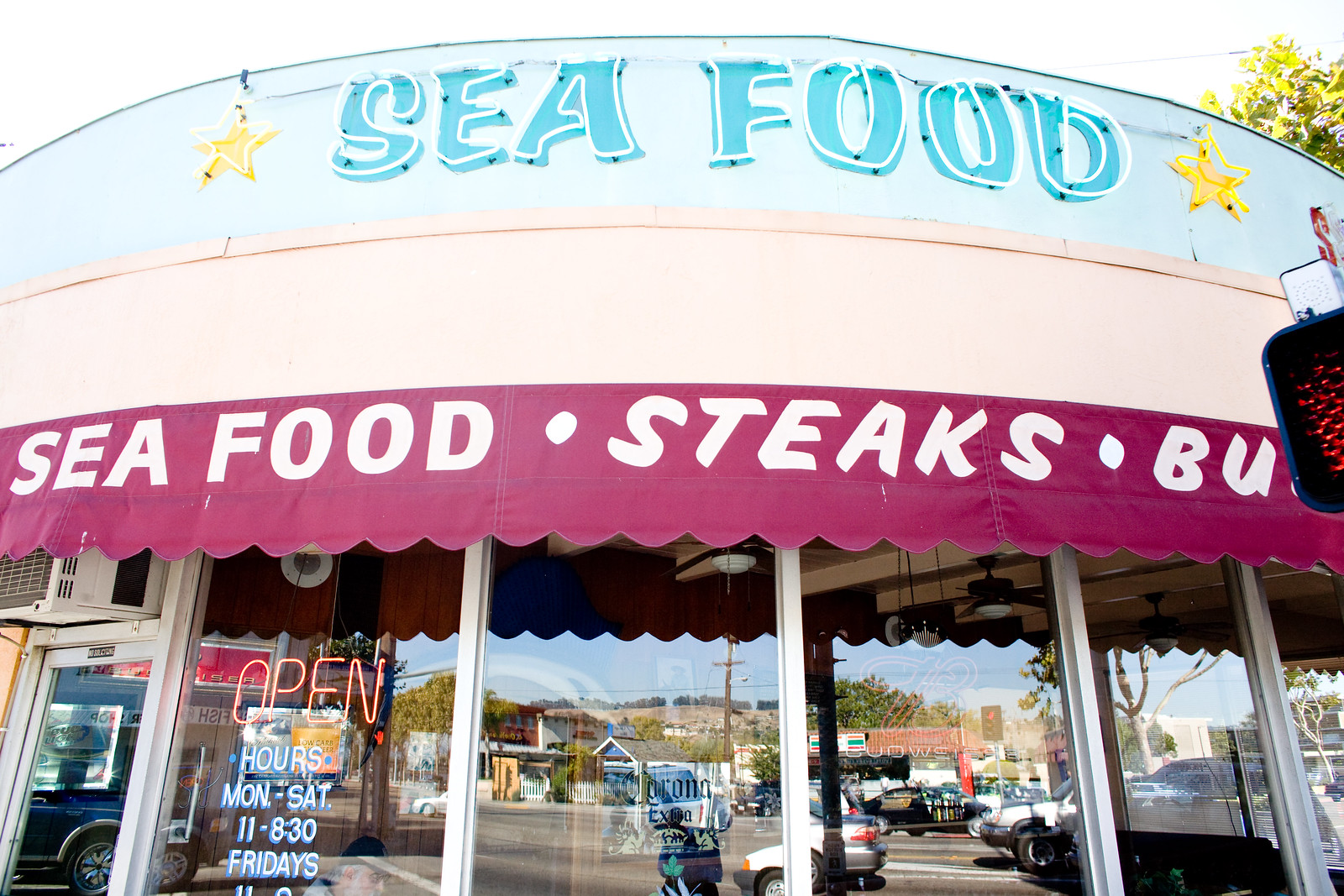This photograph depicts the front of a restaurant named "Seafood," which specializes in seafood, steaks, and burgers. The restaurant's name is displayed in prominent blue letters, flanked by yellow stars on either side of the word "Seafood." Beneath this, a smaller red banner partially shows the full menu, stating "Seafood Steaks" and likely "Burgers," though the latter word is partially obscured, only showing the letters "B" and "U." The establishment's hours of operation are Monday through Saturday from 11:00 AM to 8:30 PM, with Friday hours starting at 11:00 AM but the closing time is not completely visible. Reflections of sunlight on the restaurant's front glass reveal the words "Corona Extra," indicating that beer, in addition to the main food items, is also served. Additionally, part of a “Don't Walk” signal is visible in the image, partially cut off from the frame.